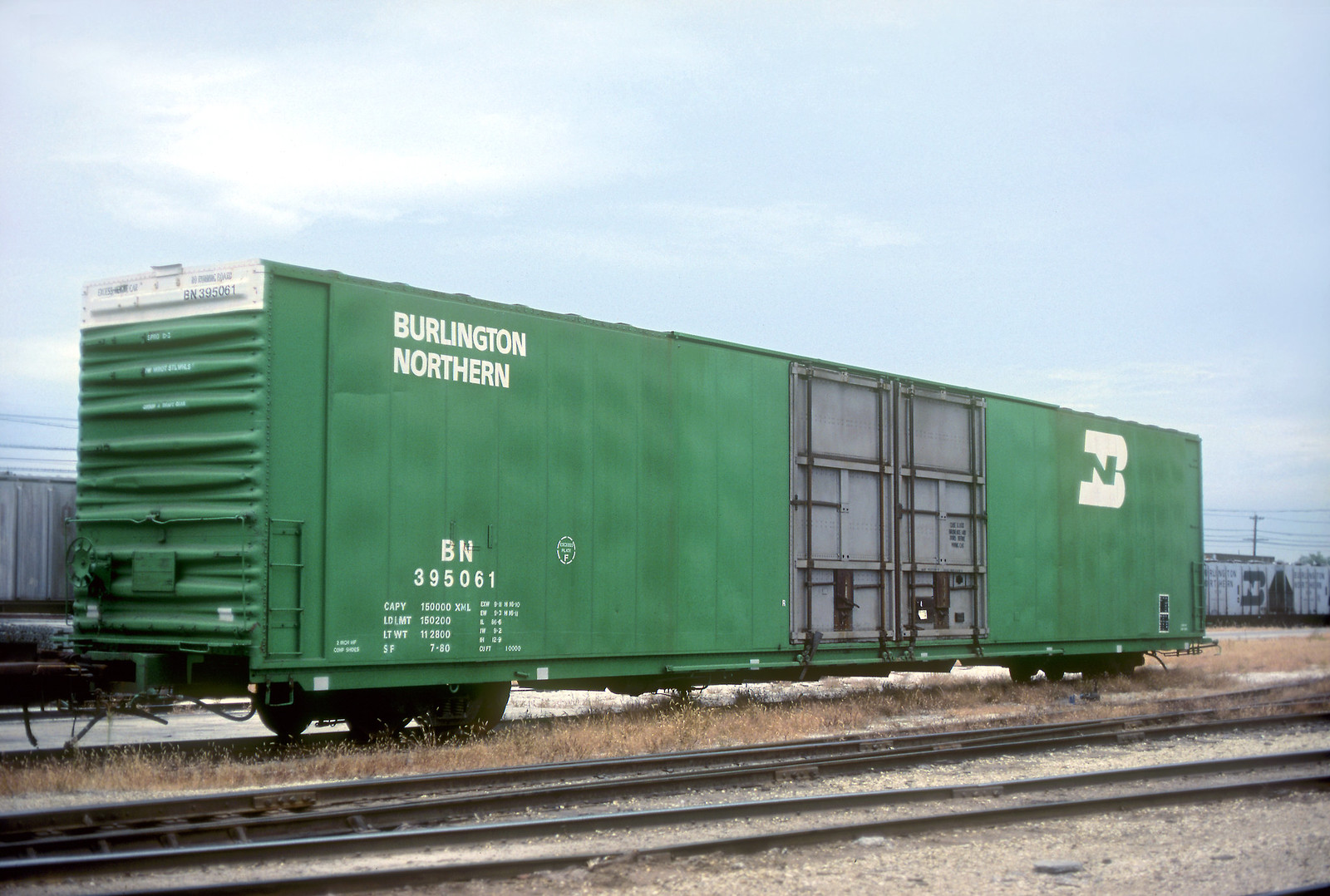The image depicts a green Burlington Northern train car, prominently featuring the white, capitalized lettering "Burlington Northern" on the left side alongside the identifier "BN 395061" below it. The Burlington Northern logo is displayed on the right side. The car has grey doors located towards the middle, equipped with black bars for additional security. Essential capacity details such as CAPY: 150,000, LDLMT: 150,200, LTWT: 112,800, and SF: 780 are visible towards the left portion of the car. Beneath the car, black wheels are supported by the tracks. The setting is an outdoor railway yard with grassy patches and additional storage cars in the background. Overhead, the sky is light blue, adorned with scattered white clouds, contributing to the serene, open-air environment of the scene.